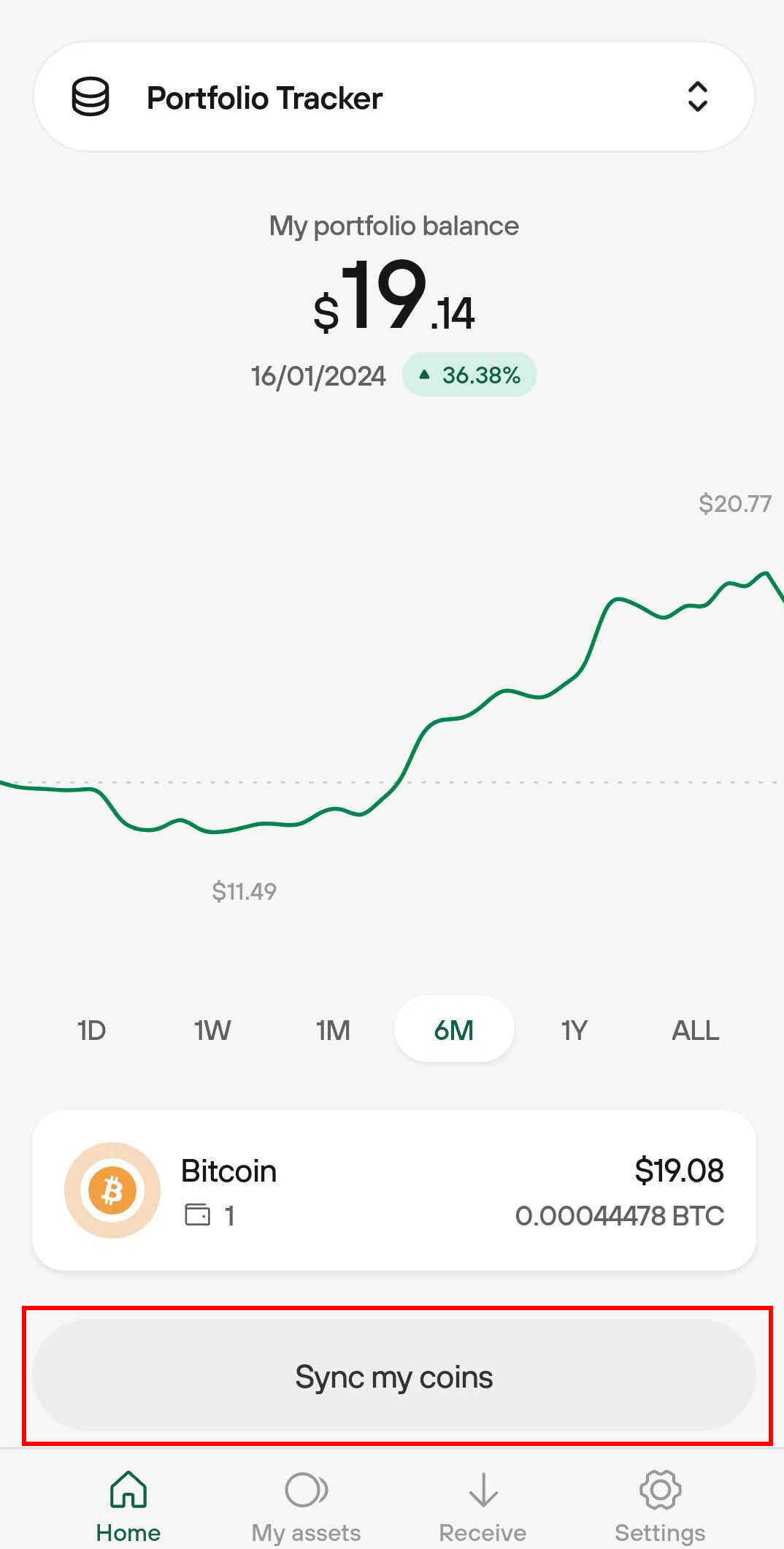The screenshot captures a mobile view of the Coinbase app. At the top, there is a search bar labeled "Portfolio Tracker," which features a black and white image of stacked coins inside the search box. Below, the header reads "My Portfolio Balance," displaying a balance of $19.14. On the top right, the performance indicator shows a green arrow pointing upwards with the amount $36.38 also in green, indicating positive performance. 

Centered below, a green line graph is highlighted, tracking the performance over "Six Months," as indicated by the white-highlighted option among the timeframes: one day, one week, one month, six months, one year, and all. Below the graph, the text "Bitcoin" is displayed with a current value of $19.08, showing ownership of 0.000044479 BTC.

At the very bottom of the screen, there is a noticeable “Sync My Coins” button enclosed by a red-edited box, indicating a user-added emphasis on this feature.